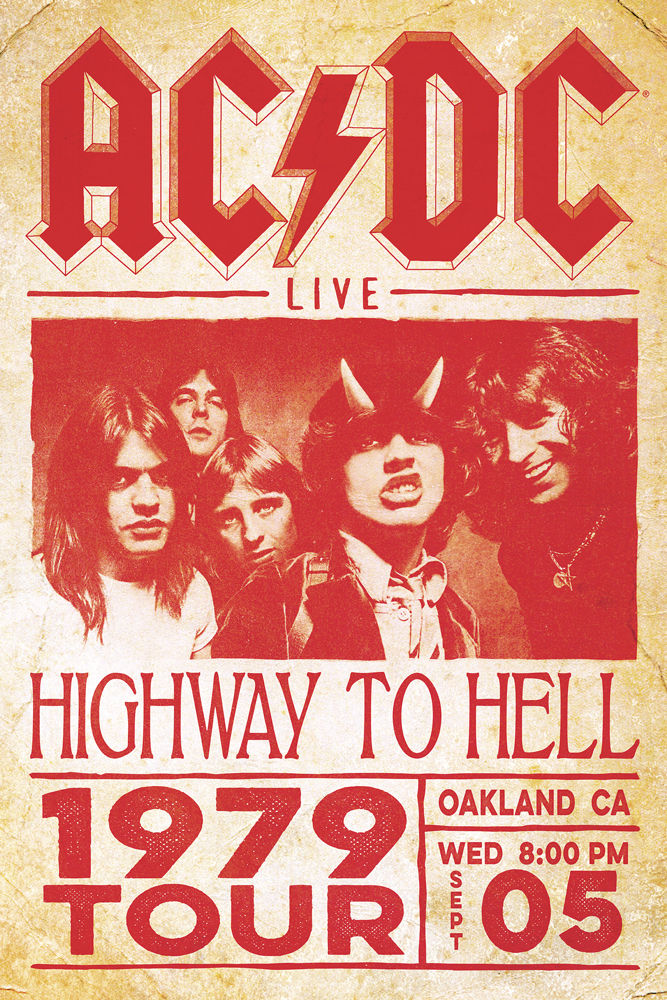This is a detailed reproduction of an old AC/DC concert poster from their "Highway to Hell" 1979 tour, specifically for their performance in Oakland, California on Wednesday, September 5th, at 8 p.m. The poster has an aged, yellowish tan background with all the text and imagery in a bold red, giving it a vintage feel. At the top, the band's iconic name "AC/DC" is prominently displayed in gothic-like letters separated by a lightning bolt. Below it, the word "Live" appears in red. The center of the poster features a boxed image of the band members—five young men, all with shoulder-length hair, staring directly into the camera. The central figure, with dark hair and a snarl on his face, wears a hat adorned with white devil horns. Beneath the band photo, the poster continues with the event details in large red capital letters: "Highway to Hell," "1979 Tour," "Oakland, CA," "WED, 8 PM," "September 05." The entire composition suggests a collectible quality, suitable for framing and display, devoid of any visible creases, further indicating that this is likely a reproduction.